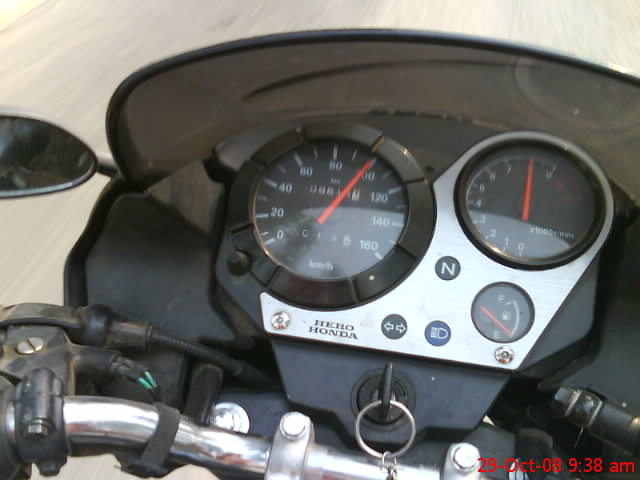Date stamped "29-October-08, 9:38 AM" at the bottom right, this action shot captures the dynamic view of a motorcycle dashboard in motion against a grey, water-lined ground. The left side features a speedometer marked in kilometers per hour with a red needle pointing to 100 km/h, on a scale ranging from 0 to 160 in increments of 20. To the right, an RPM gauge reads at 8, signifying 8,000 RPM on a scale from 0 to 9.

The dashboard is branded with the Honda logo and hosts several controls and indicators. A silver button is on the left, and a black circle on the right displays left and right turn signals along with a headlight symbol, designed as a sideways "D" with dashes to the left. A black circle with a white "N" indicates neutral, and to its right is a fuel gauge showing levels from empty to full, with a red indicator needle. Central to the dashboard is the ignition key encircled by a silver ring.

Barely visible in the shot are elements like a sturdy silver bar with bolts at both ends running across the bottom left, and a handlebar on the left featuring a modest black screw. The left side view mirror is also visible but does not reflect any scenery. The entire dashboard is sheltered by a transparent windshield, encapsulating the rider's perspective.